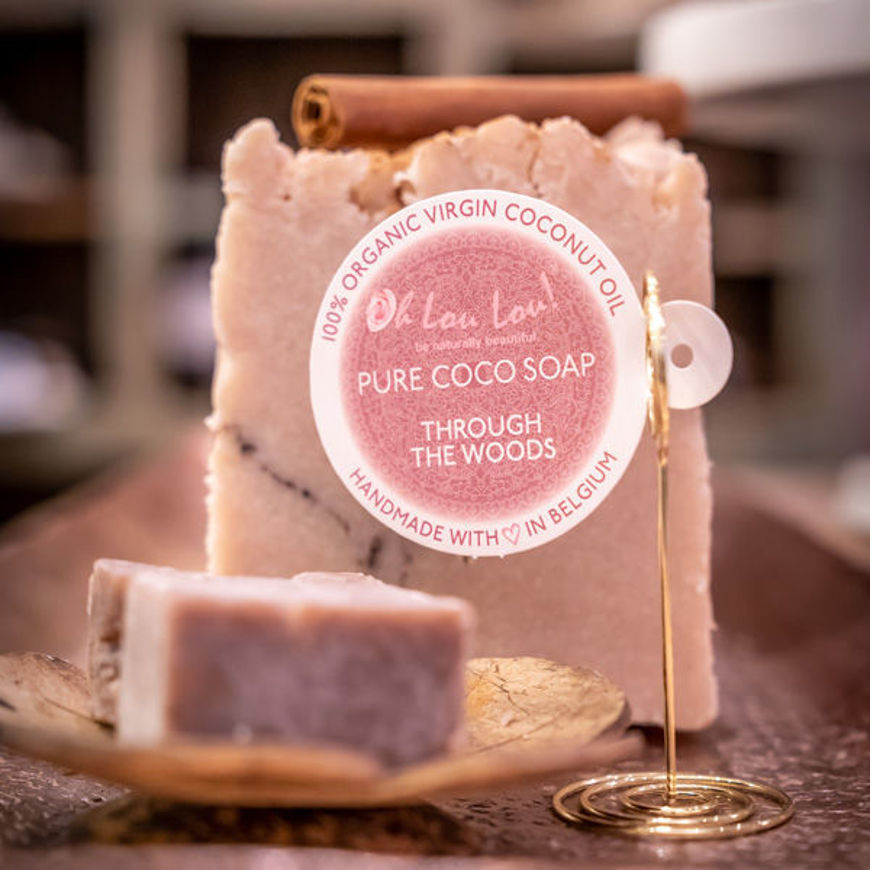This close-up image showcases a meticulously crafted bar of soap on display, framed by a distinctive brass sign holder. The brass holder features a spiral circular base, a vertical pole, and another spiral circular support from which a circular disc-shaped sign hangs at a 90-degree angle. The sign prominently reads "Pure Cocoa Soap" and "100% Organic Virgin Coconut Oil," further adorned with "Oh La La! Pure Cocoa Soap Through the Woods Homemade with Love in Belgium." The somewhat out-of-focus bar of soap in the background is a warm tan color with delicate black striations. Resting on top of the soap is an elegantly placed cinnamon stick, adding a rustic and wholesome touch to the presentation. The intricate details of the sign holder and the natural elements combined create a charming, artisanal display.